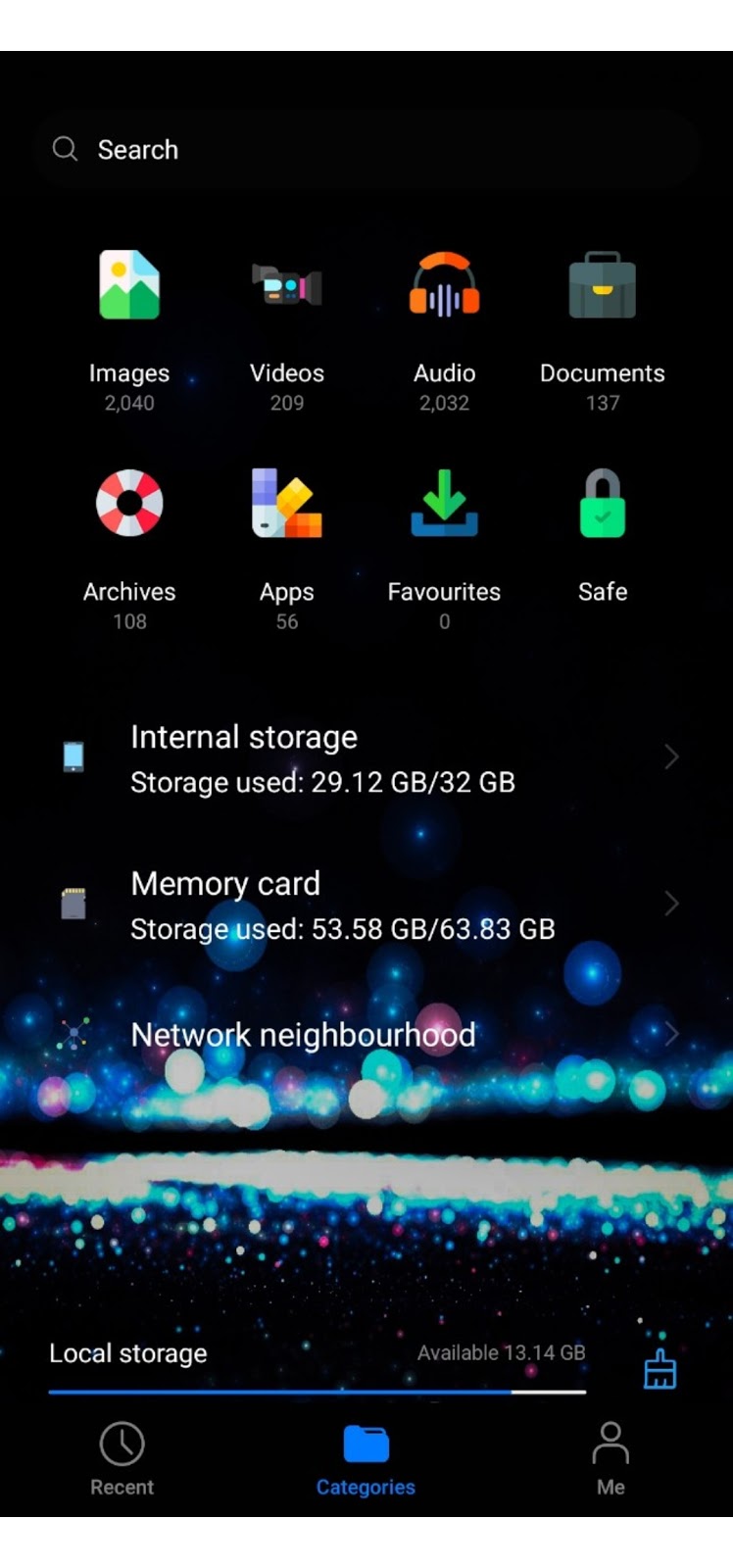This image is a vertically oriented mobile screenshot featuring a user interface with a jet black background. At the bottom, there's an abstract, colorful bubble design in shades of blue, magenta, and light blue.

At the top-left corner, there's a search icon accompanied by the word "Search." Eight icons are organized into two rows beneath this. The first row includes icons labeled: Images, Videos, Audio, and Documents. The second row includes icons labeled: Archives, Apps, Favorites, and Save.

Centrally located, there are two parts labeled "Internal Storage" and "Memory Card." For "Internal Storage," 29.12 GB of the available 32 GB are used. For "Memory Card," 53.58 GB of the available 63.83 GB are used. Below this, the interface references "Network Neighborhood."

At the footer of the screen, there is a blue slider bar representing local storage usage, almost fully filled. To the left of the slider bar are three icons labeled Recent, Categories, and Me, with the Categories icon and text highlighted in blue. A blue paintbrush icon is located at the right-hand side of the slider bar.

This detailed interface provides a comprehensive view of storage management and quick access to various file categories.